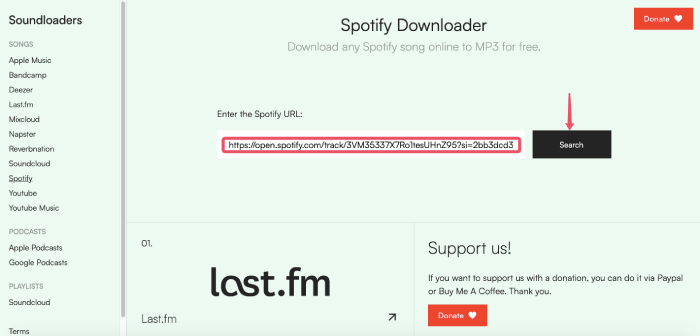The image showcases the user interface of the Spotify Downloader website. The main section features a prominent text box where users can enter the Spotify URL of the song they wish to download, such as "https://open.spotify.com/track/3VM35337X7ROR1ESZJHNZ9?si=2BB3DEDE3". Below this text box, there is a "Search" button that initiates the download process.

Key features of the site include the ability to download any Spotify song as an MP3 file for free. The interface encourages users to support the service through donations, with options like PayPal or "Buy Me a Coffee," and a convenient "Donate" button is provided.

On the left side of the screen, a navigation menu lists various platforms for downloading songs and podcasts, including Apple Music, BandCamp, Deezer, Last.fm, Mixcloud, Napster, Soundcloud, Spotify, YouTube, and YouTube Music, as well as potentially ReverbNation. There might also be links for terms and additional options, though they aren't clearly visible in this summary.

The design is straightforward, focusing on functionality and ease of use, with additional sections for affiliate links like Last.fm. It's mentioned that Last.fm is still in use by some people, though its current status is uncertain. Finally, there is a disclaimer questioning the legality of the service and its current availability.